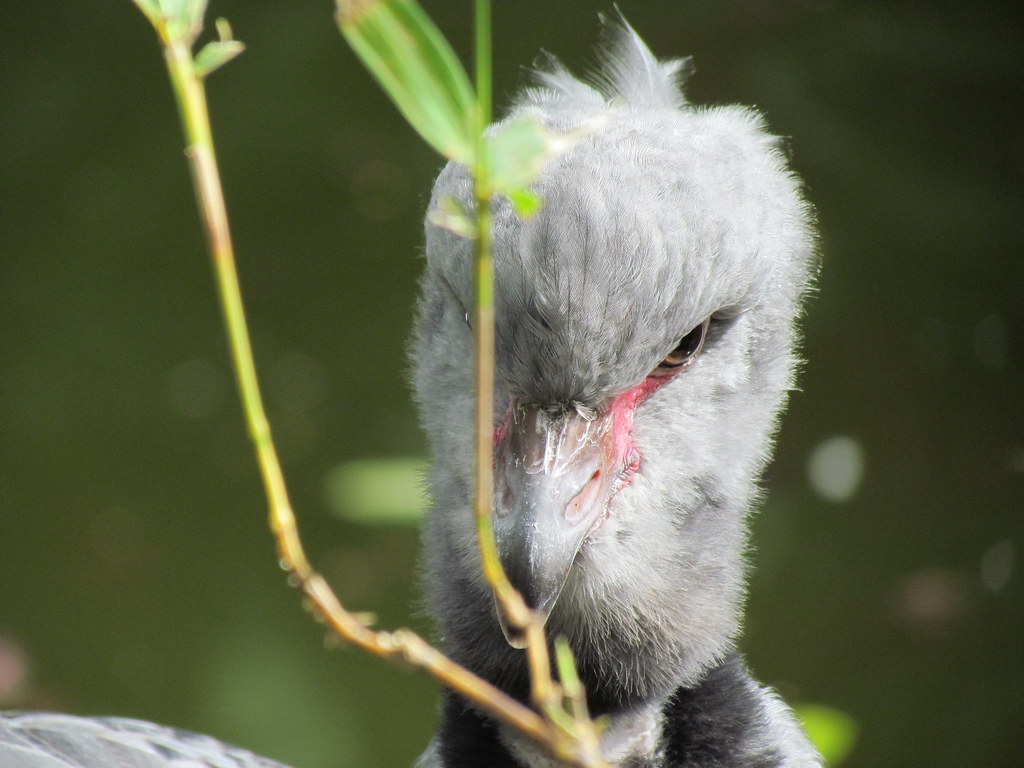In this close-up image, positioned against a dark olive green, blurry background, the focal point is the head of a young bird. The bird's head is predominantly covered in fluffy, whitish-gray feathers, giving it a soft and fuzzy appearance. The neck features a distinctive black and white V-shaped pattern. The bird's beak is a mix of light gray and black at the tip, with a hint of pink extending from the eye to the beak. Only the bottom edge of its right eye is visible, showing the pink area near the tear duct. In the foreground, there are blurry green and brown branches extending from the bottom to the top of the image and one green leaf adds a touch of color to the composition. The bird's head appears slightly tilted downward, contributing to the gentle, detailed focus on its delicate features.